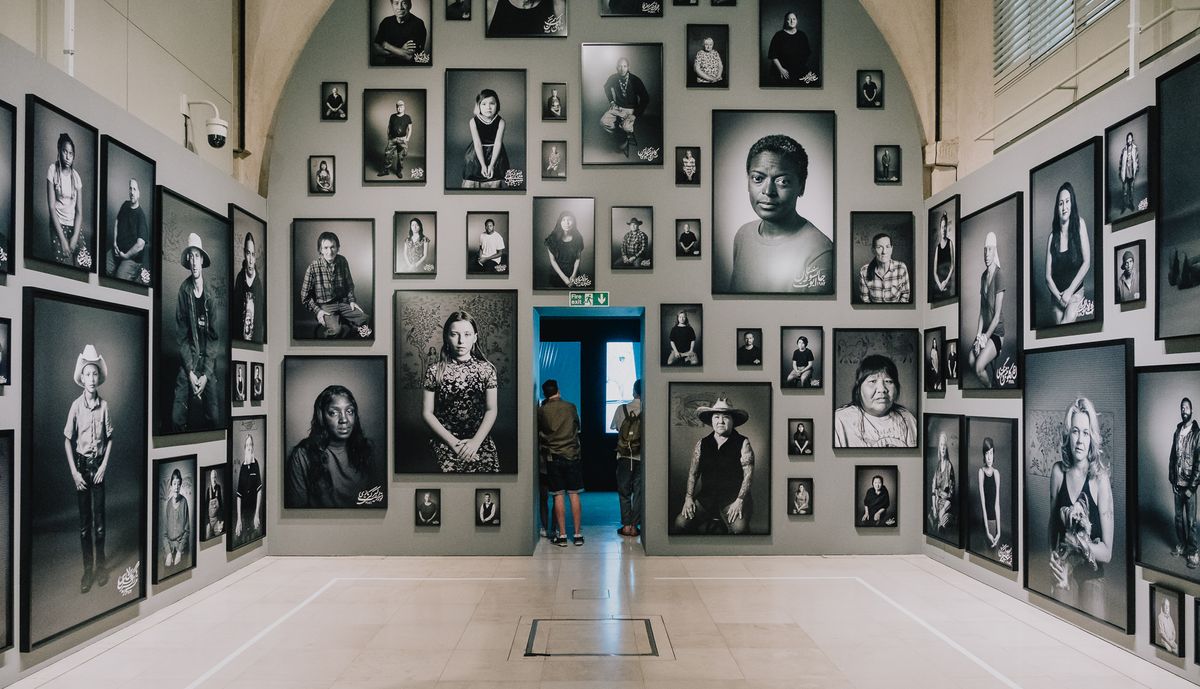This photo captures an interior space that resembles an exhibit hall or museum gallery, characterized by its high ceiling and white flooring. The walls, predominantly white and gray, are adorned with an extensive array of 40 to 50 black and white portraits, showcasing a diverse range of people from various ethnic backgrounds, ages, and walks of life. These portraits include young children, young adults, and older individuals, encompassing different characters such as cowboys and Native Americans. Each subject appears to be posed rather than candid, creating a formal atmosphere. The portraits are arranged on all visible walls—right, left, and background—with the sepia-toned and grayscale images providing a sense of historical diversity. Notably, on the lower left, a young boy is dressed as a cowboy with a hat and jeans, while other images depict young girls with pigtails and elderly women in shawls. In the center of the room, there is an entrance to another area characterized by its blue floor and wall. Two people stand in this doorway—one wearing a backpack, the other sporting shorts and running shoes—seemingly engaged with the display beyond.